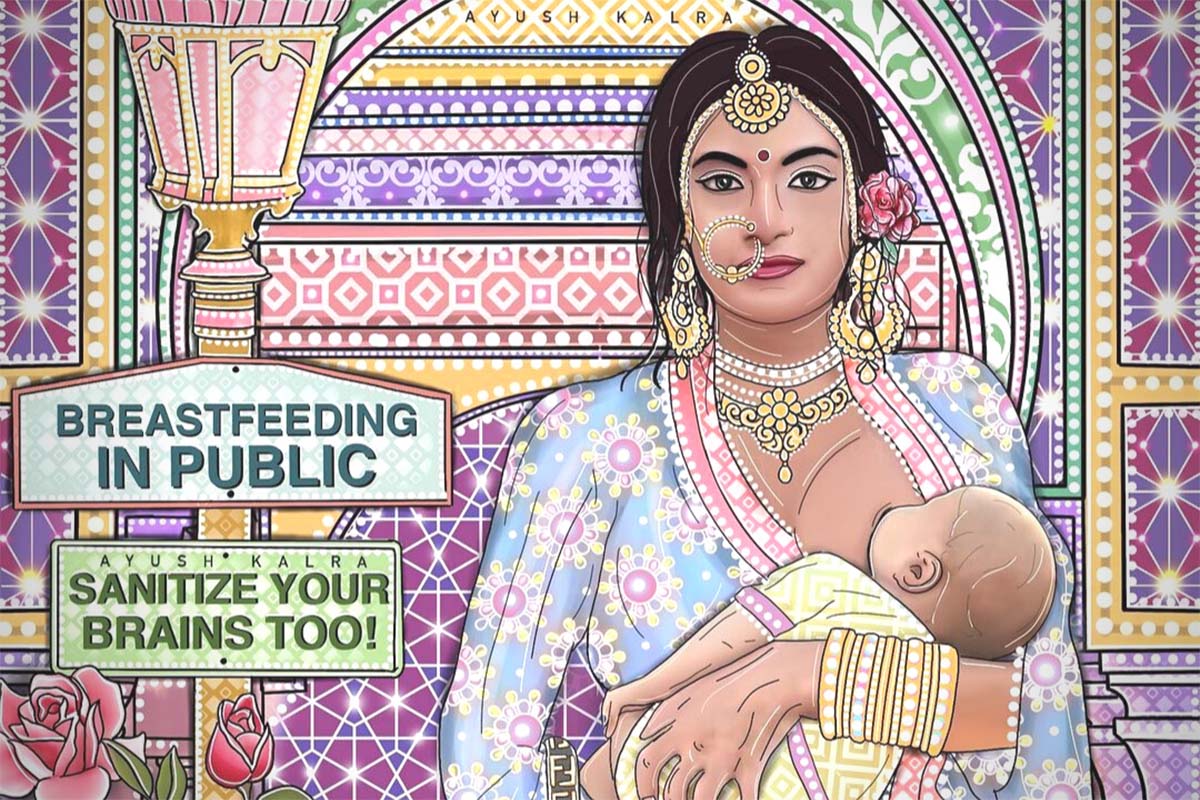This advertisement, likely a public service announcement, features a detailed and colorful drawing of an Indian woman in a landscape layout. Positioned on the right, the woman—recognizable by her traditional attire and adornments—is in the act of breastfeeding her baby. She has long dark hair, embellished with golden pearls and a rose behind her ear. Her accessories include a prominent circular gold nose ring, dangling gold earrings, a bindi on her forehead, and a multitude of bracelets on her left arm. 

The woman is dressed in a vibrant blue and purple floral dress with accents of pink and yellow, and she wears a gold and white necklace. The baby she cradles, feeding at her exposed left breast, is clad in a yellow and pink outfit. 

The left side of the image features a golden pole with a sign that reads, "Breastfeeding in Public," followed by the message, "Sanitize Your Brains, Too," and the name "Ayush Cholera." The background is richly decorated with an array of bejeweled designs, incorporating an Easter color palette of purples, pinks, yellows, and greens, which complements the woman’s attire and the overall aesthetic of the illustration.